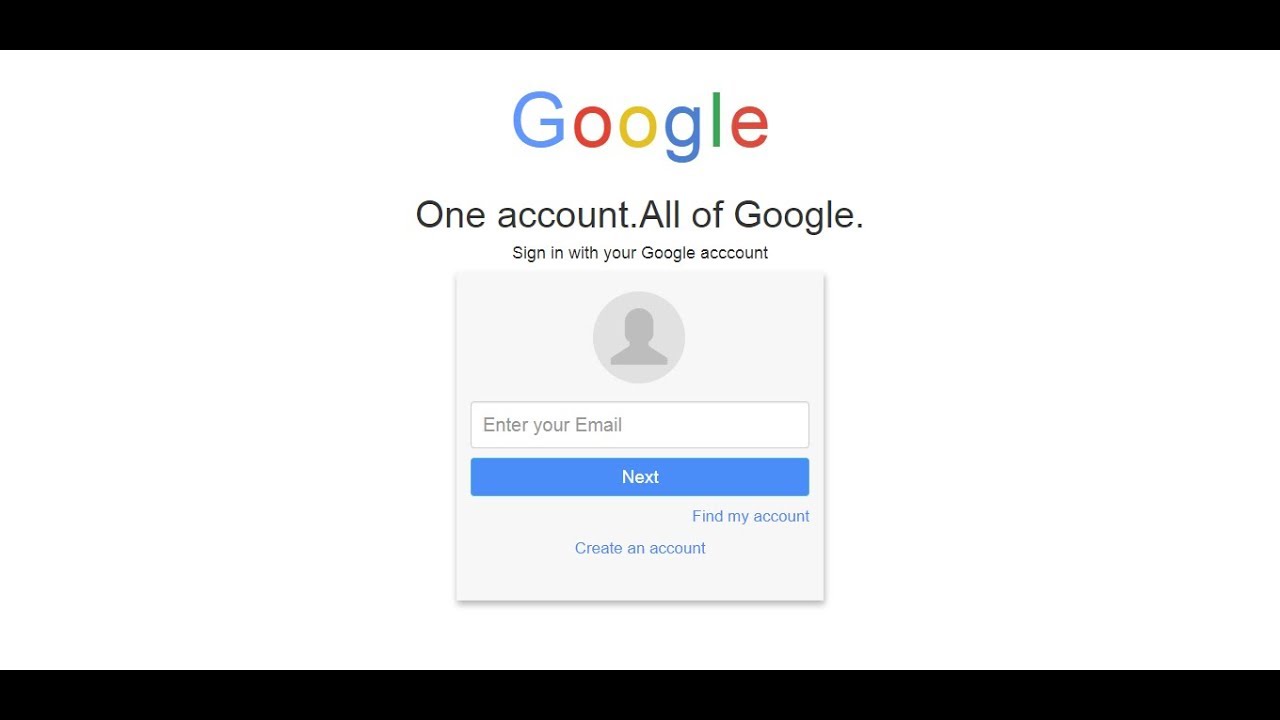The page features an unmistakable Google branding showcased through its balanced and simple design. At the very top and bottom of the page, there are long, narrow horizontal black bars acting as borders, which frame the central content against a clean, white background. 

The focal point near the top of the page is the Google logo, composed of the iconic multi-colored letters: a blue "G," a red "O," a yellow "O," a blue "G," a green "L," and a red "E." Directly beneath this vibrant logo is the tagline written in concise black text: "One account. All of Google." This succinctly conveys that a single login grants access to the myriad of Google services.

Below this tagline, in smaller black text, is a prompt encouraging users to "Sign in with your Google Account." This leads to the primary function of the page: account login.

Next, users are presented with a gray box meant for entering their credentials. Inside this box, there's a placeholder where a user’s profile picture would typically appear, represented by a grayed-out, circular avatar devoid of any photo. Just below this is a text box labeled "Enter your email," inviting users to type in their email address.

Following this input field, a prominent blue rectangular button labeled "Next" encourages users to proceed after entering their information. Beneath this button, a blue hyperlink reads "Find my account," providing assistance for users who might have forgotten their login details. Finally, at the bottom of the section, another blue hyperlink states "Create account," guiding new users towards account creation.

The design is minimalistic and user-focused, streamlining the navigation towards either account recovery or creation.